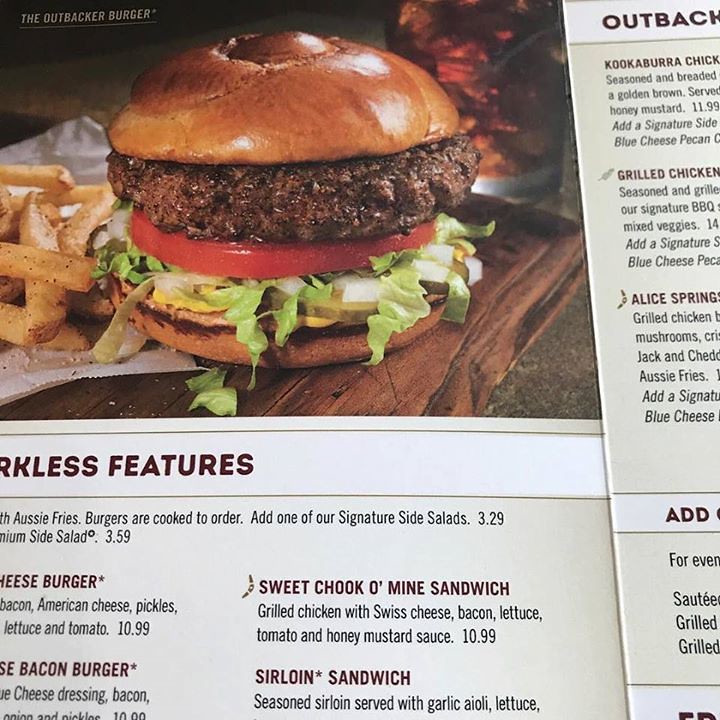**Detailed Caption:**

The image depicts a section of the Outback Steakhouse menu, prominently featuring the "Outbacker Burger" in the upper left corner. The name "Outbacker Burger" is displayed in all capital letters with white lettering, accompanied by a horizontal line underneath. Adjacent to the line is a registered trademark symbol (®). The burger is visually highlighted, showcasing a hearty patty topped with fresh tomato slices, crisp lettuce, and tangy pickles. The burger bun appears unique, possibly featuring a special texture or design. Accompanying the burger to the left are seasoned fries, adding a flavorful side to the meal. To the right of the burger and fries, there is a clear glass filled with a cold drink and ice, suggesting a refreshing beverage to complement the meal.

Beneath the image of the burger, there are partially visible words and phrases describing menu items and features, such as "Aussie fries," "add more to your side," "cheeseburger," "bacon burger," and "sirloin sandwich." Among these, an intriguing item is mentioned: the "sweet choke oatmild sandwich," which likely denotes a sandwich with a unique combination of ingredients. The right-hand side of the image slightly shows a portion of the next page of the menu, hinting at additional offerings and continuing the array of tempting dishes available at Outback Steakhouse.